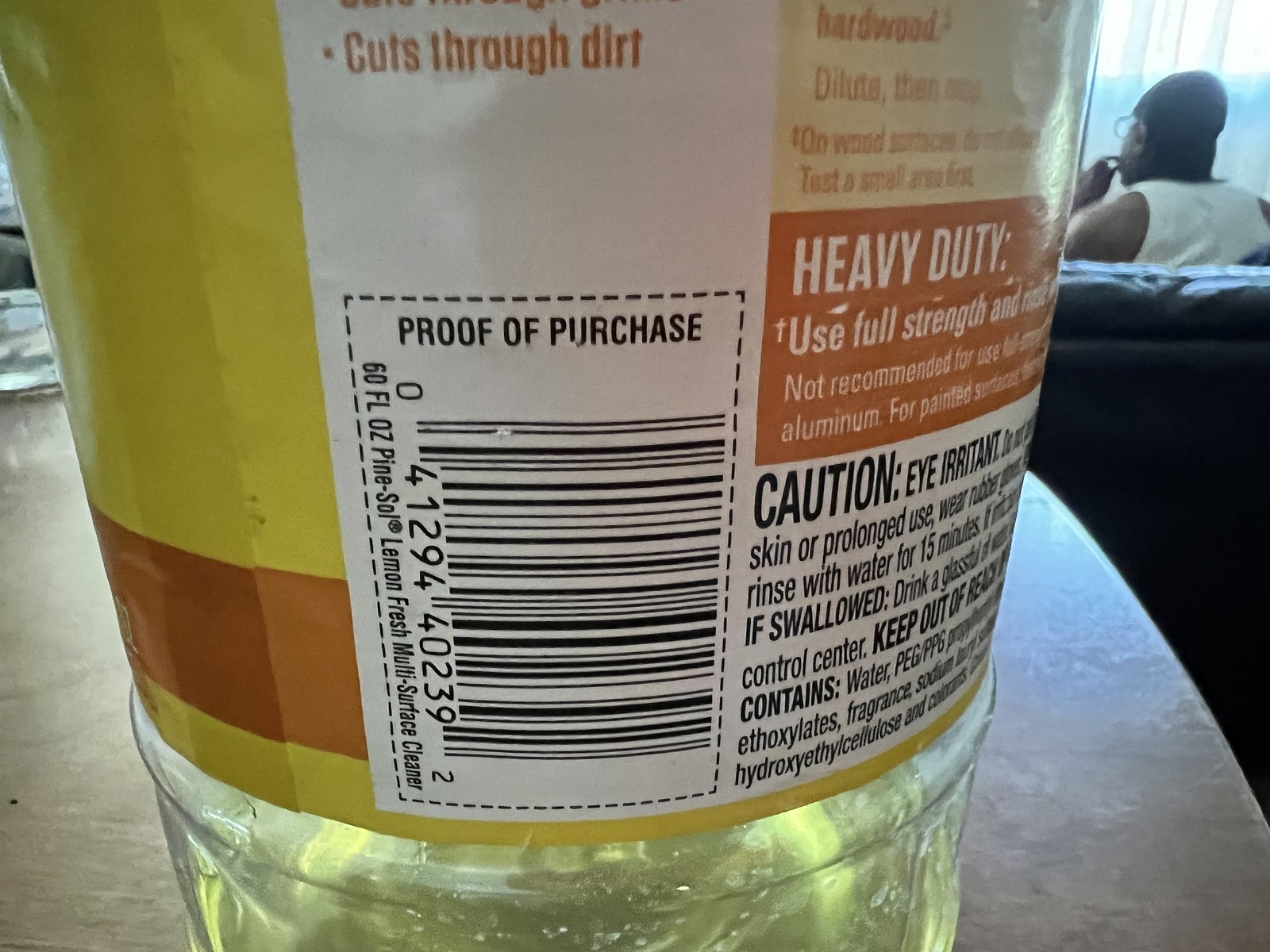The image shows a close-up of a plastic bottle containing a yellow liquid, identified as Pine-Sol Lemon Fresh Multi-Surface Cleaner. The bottle, marked with a proof of purchase and a barcode, holds 60 fluid ounces. In an orange section of the label above the barcode, the words "Cuts Through Dirt" are prominently displayed. The label also contains warnings such as "caution eye irritant" and instructions on what to do if swallowed, along with a directive to "use full strength" for heavy-duty cleaning. The background features a wooden table on which the bottle sits, with a black couch behind it. A dark-complexioned man with glasses and a white tank top is visible, facing away from the camera. Sunlight filters through a window with a curtain, adding a natural light element to the scene.